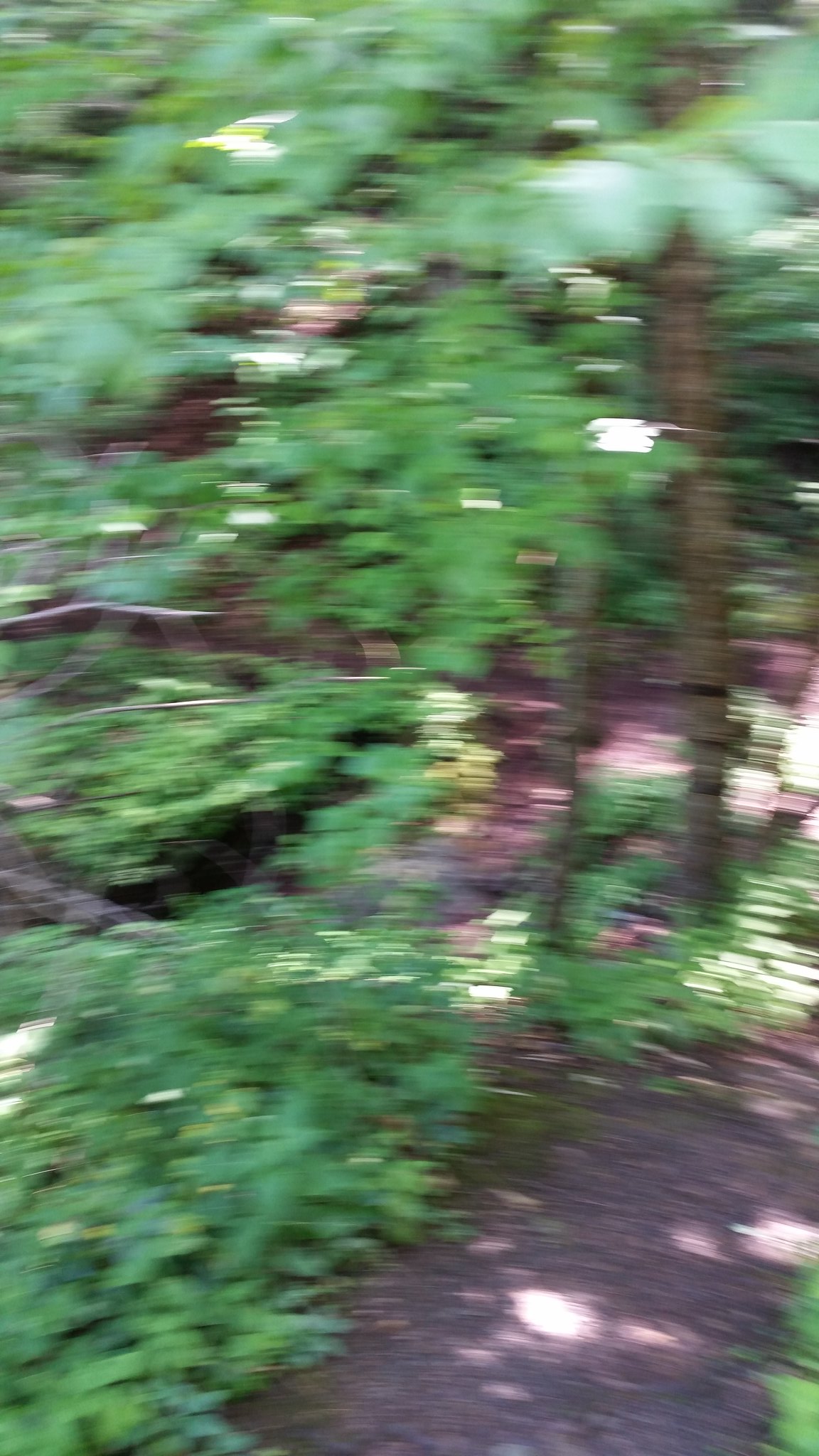This photograph captures a densely wooded area, potentially a walking trail within a forest. The image appears blurred, likely due to the photographer’s movement, suggesting either haste or excitement at the moment. The scene is dominated by a variety of trees with plentiful lush vegetation, hinting at a verdant, thriving ecosystem. A dirt path can be discerned winding through the trees, characteristic of many forest hiking trails. The photograph is somewhat zoomed in, making it difficult to pinpoint the exact location, but it evokes the tranquility and natural beauty often found in national parks or similar nature reserves. There are no people, animals, or text present in the image, allowing the viewer to focus solely on the serene forest environment.